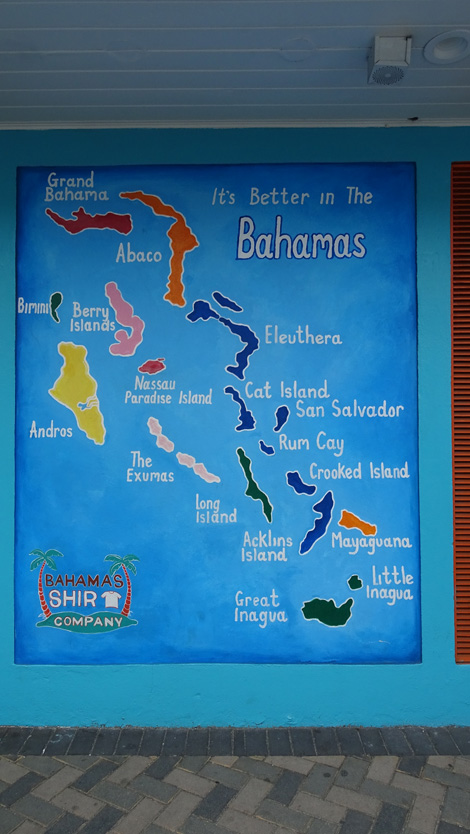This image features a large, detailed mural of a map of the Bahamas, painted on an exterior wall. The mural stretches from about a foot above the concrete interlocking brick walkway at the bottom to approximately a foot below the ceiling at the top. The map has a vibrant blue background symbolizing the surrounding water, with various islands depicted in a range of colors including red, orange, yellow, green, blue, and peach. Each island is individually labeled in white text, showing names like Grand Bahama, Abaco, Berry Islands, Cat Island, San Salvador, Andros, and many others.

Prominently positioned in the top right corner is the phrase "It's Better in the Bahamas." At the bottom left of the mural, between two palm trees, is a logo with the text "Bahamas Shirt Company." Notably, the 'T' in 'Shirt' is creatively replaced with an illustration of a T-shirt, reinforcing the theme. The mural effectively captures the geographical essence and colorful spirit of the Bahamas.